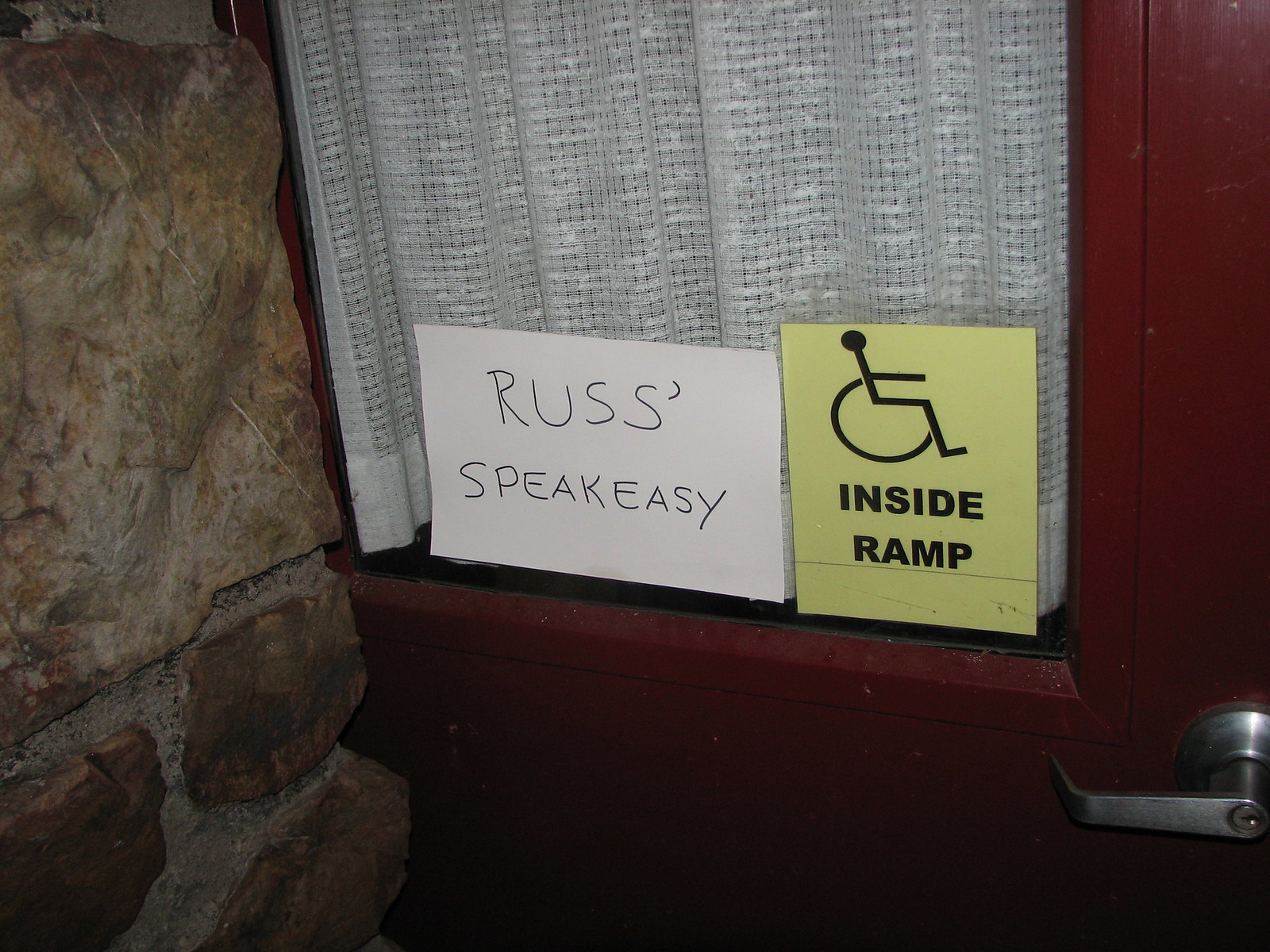This large, square photograph captures an old-fashioned wooden door set into a stone wall composed of both large stones and smaller bricks connected by mortar, with noticeable newer grouting. The door, a rich dark cherry wood, features a window framed on the left side adorned with a semi-transparent white lacy curtain. In the window, there are two signs: a handwritten white sign that reads "Russ's Speakeasy," and a smaller, vertically rectangular yellow sign featuring a wheelchair icon with the words "Inside Ramp" in bold black letters beneath it. The bottom right corner of the door displays a long, silver handle with an integrated keyhole. The image has a slightly dark ambiance, especially towards the lower part of the door, suggesting lower lighting in this area.